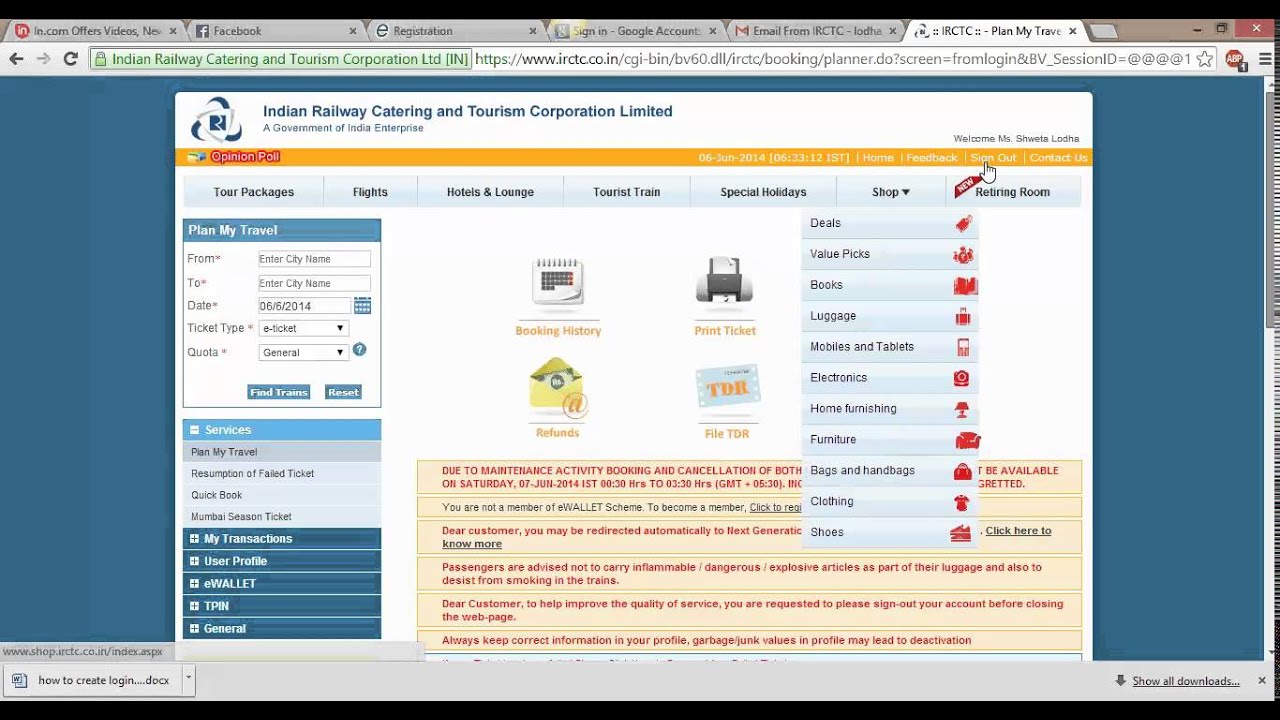A detailed screenshot from a Windows operating system browser window displays six open tabs. The browser could potentially be either Explorer or Chrome.

1. The first tab, marked with a red circle containing "IN," partially shows the title "IN.COM offers videos,..." followed by an unreadable section.
2. The second tab is for Facebook.
3. The third tab presents a large letter "E" and mentions "registration."
4. The fourth tab is a Google account sign-in page, displaying an open Gmail with an email from IRCTC.
5. The fifth tab is the IRCTC website, labeled "IRCTC Plan My Travel." Below it, the full name, "Indian Railway Catering and Tourism Corporation Limited," is shown, indicating it's a government enterprise of India.

The IRCTC website has a comprehensive interface:
- It includes options to purchase tickets, highlighted by specifics such as selecting the departure and destination points, travel date, ticket type, and quota.
- There is a visible yellow opinion poll dated June 2014.
- Navigation buttons include Home, Feedback, Sign Out, and Contact Us.
- The site offers various services, including tour packages, flights, hotels, tourist trains, and special holidays.
- The current selection is under the "Shop" drop-down menu featuring categories like deals, value picks, books, luggage, electronics, home furnishings, furniture, bags, clothing, and shoes.
- A new section for booking retiring rooms is indicated with a "New" tag.

The detailed IRCTC site is designed for user convenience in planning and booking travel as well as purchasing additional items from the shop section.